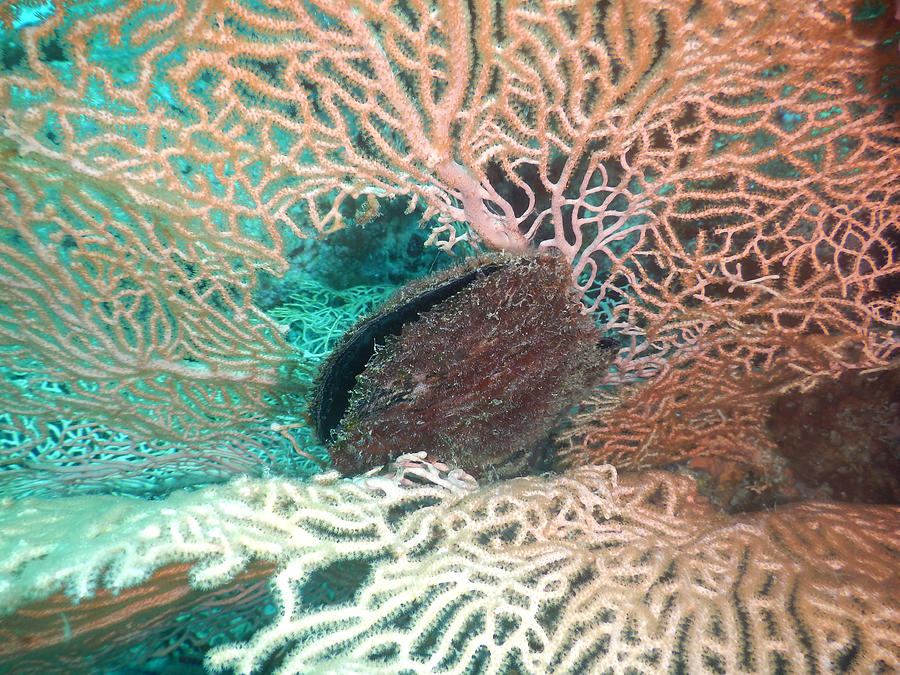This underwater photograph captures a mesmerizing marine scene featuring diverse sea life. Central to the image is a furry brown structure resembling a sea urchin or an intricate coral cluster, with net-like white and brown patterned tentacles radiating from it. Surrounding this central form is a vivid array of crenulated corals, exhibiting a wavy texture reminiscent of brain coral. The corals vary in color, including shades of blue, beige, orange, and brown, with fine, sharp edges. The bottom of the image prominently features white coral, while the deep blue water forms the serene backdrop. Off to the right side, another brown element is visible, adding to the rich palette of natural hues captured in this exquisite underwater nature photograph.